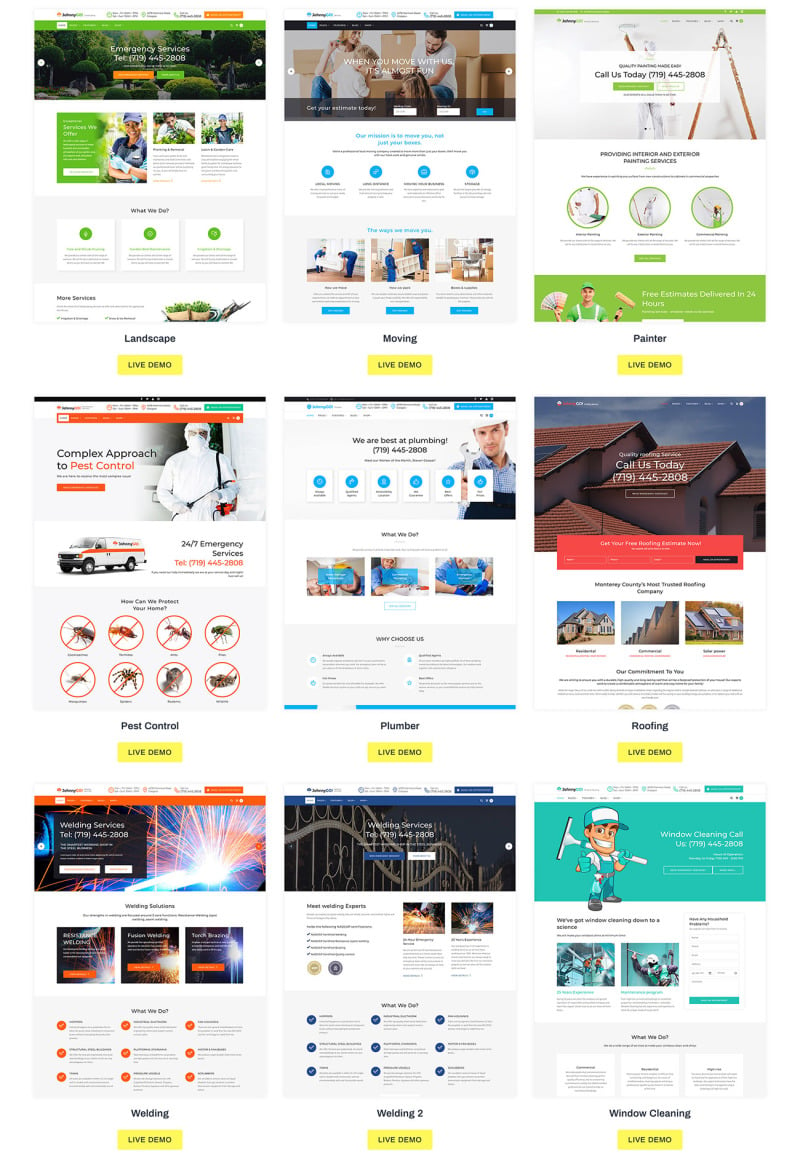The screenshot features multiple images set against a white background, each accompanied by white squares containing information. Here's a detailed breakdown of the elements in the screenshot:

1. **Mountain and Forest Image**: The first image showcases a picturesque mountain scene that transitions into a dense forest. Below this image, there are three white squares neatly arranged, each containing some textual information.

2. **Man and Woman with Moving Boxes**: The second image depicts a man and a woman in the process of moving. Numerous boxes clutter the scene, suggesting a relocation. Like the first image, this one is also accompanied by three white squares with information.

3. **Ladder Image**: This image simply features a ladder, possibly indicating a step-by-step process or a guide. Adjacent to the ladder, there are three white squares with text, providing further details related to the image.

4. **Pest Control Image**: A man dressed in all white stands prominently in this image. The text "Pest Control" is emblazoned in orange next to him. Surrounding this text are eight circles, each depicting a different type of bug, all with slashes through them, indicating extermination.

5. **Construction Worker Image**: Another image features a man wearing a hard hat and a blue shirt, suggesting he is a construction worker. This image is complemented by six white squares that contain relevant information.

6. **House Image**: The final image in the screenshot shows a house. Like the previous images, it is augmented by three white squares with text that provides additional context or information.

This descriptive caption aims to clearly convey the visual and textual elements present in the screenshot, providing a comprehensive overview for the viewer.